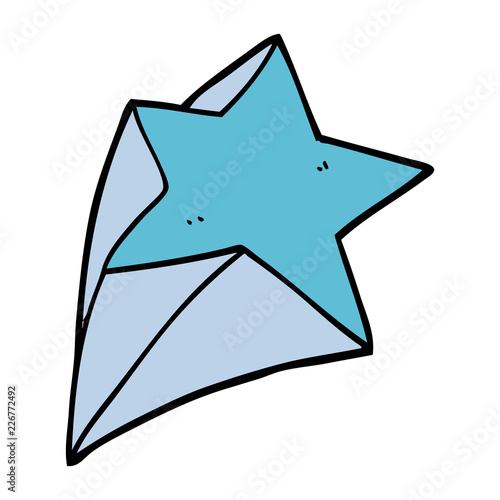This image features a three-dimensional, aqua-colored star with a trailing tail, suggestive of a shooting star, rendered in shades of blue and lavender. The star, centrally positioned against a white background, is outlined in black. Its long tail, fading in color, extends diagonally from the bottom left to the top of the image. Over the entire image, a transparent watermark with the text "Adobe Stock" appears repeatedly. In the lower left corner, in black vertical text, the identifier "Adobe Stock" and the stock number "226772492" are also present, indexing the image for easy referencing.